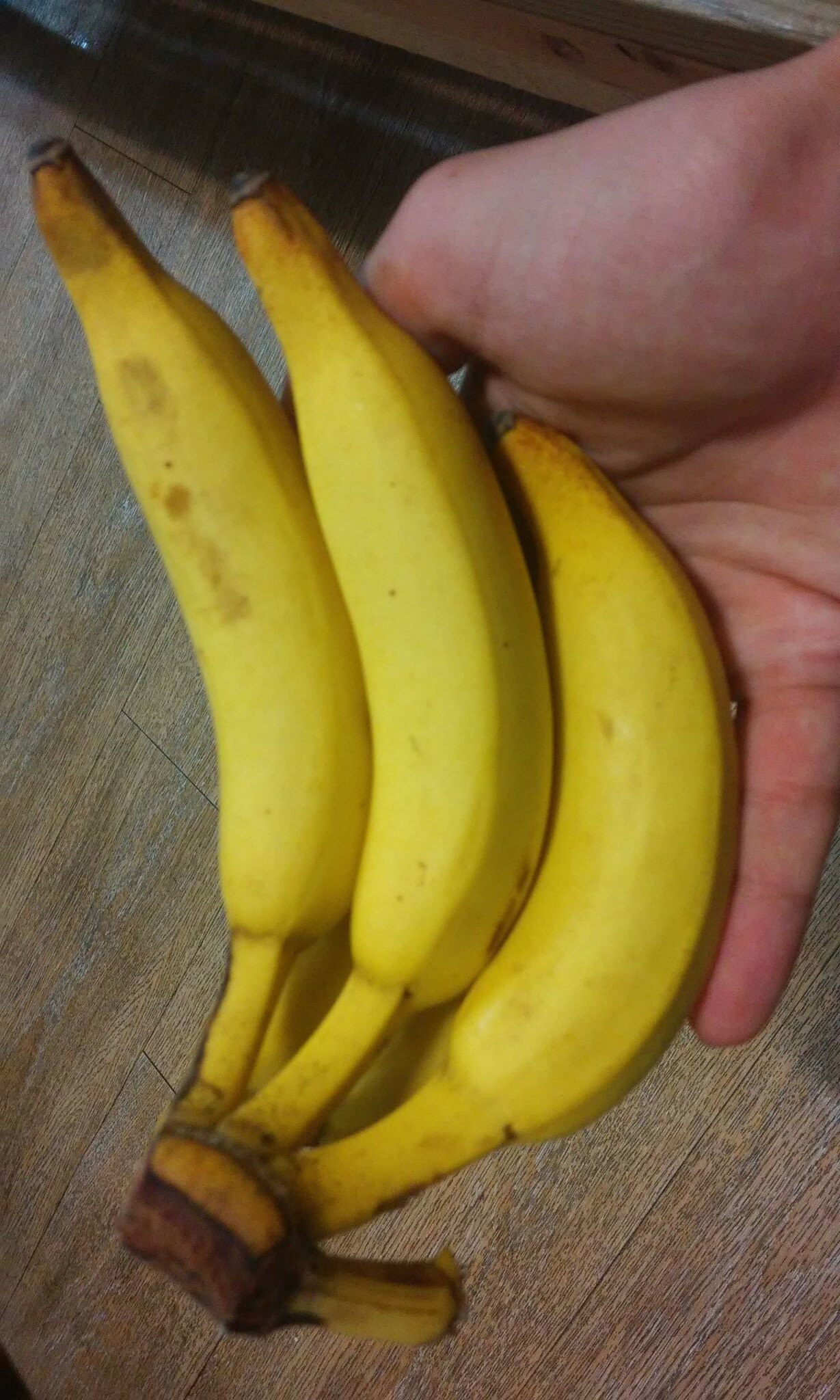This overhead photograph captures a ripe bunch of three bananas being held by a person's right hand, the palm facing upward. The bananas, notably yellow with slight browning and black spots at the tips, rest on a light brown wooden floor with pronounced grain and high contrast. The hand, which appears to be Caucasian, shows a missing banana from the cluster, indicated by an empty stem. The image is taken from a diagonal aerial perspective, adding a dynamic slant to both the bananas and the wooden background below them.